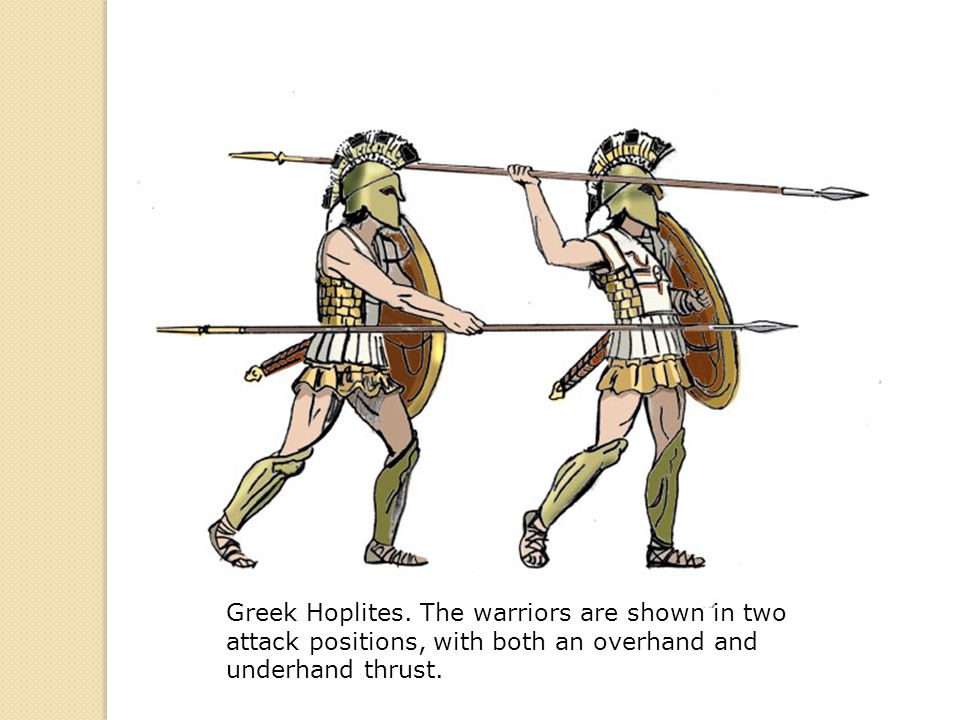This detailed illustration, reminiscent of a textbook or encyclopedia page, depicts two Greek hoplites in battle attire. The image features side profiles of the warriors, who are seen wearing golden helmets adorned with feathers, chain mail tunics, shin guards, and sandals. Each hoplite wields a round shield and a long spear. The text beneath the image reads, "Greek hoplites. The warriors are shown in two attack positions with both an overhand and underhand thrust." The hoplite in the foreground employs an underhand thrust with his spear, his arm extended forward, while the hoplite in the background utilizes an overhand thrust, his spear raised above his shoulder. The craft of the illustration, combined with its textbook placement, provides a detailed view into the military attire and combat stances of ancient Greek warriors.